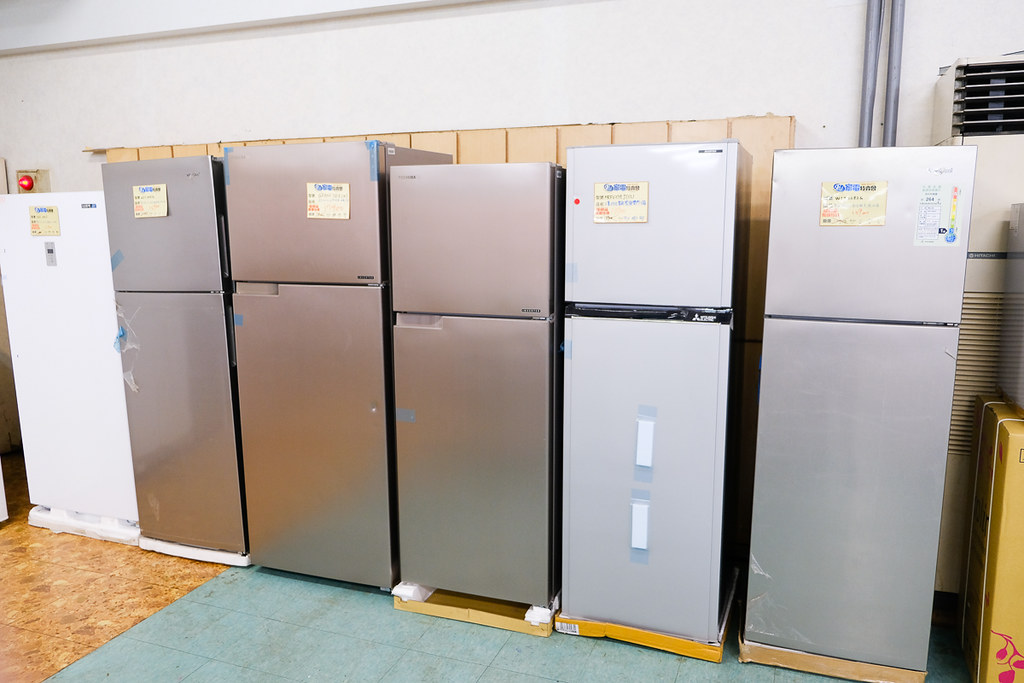This photograph captures a row of six vertically-standing refrigerators, likely taken in a store or warehouse setting. The image features various models of fridges, including a mix of white and stainless steel units, all with freezers on top. From left to right: 

1. A single-door white refrigerator on a white pallet.
2. A slightly taller single-door stainless steel refrigerator, with about 60% of its height dedicated to the fridge section and 40% to the freezer, also on a white pallet.
3. A stainless steel refrigerator of similar style with a rectangular handle cut out on the top left corner of the lower door, slightly taller and on a cardboard box.
4. Another stainless steel refrigerator matching the style of the previous unit but slightly shorter.
5. A white refrigerator with the same 60%-40% split, also on a cardboard box.
6. A final stainless steel refrigerator with the same proportions and on a cardboard box.

The floor beneath the first two fridges appears to be a wood-like tile, transitioning to an off-white gray tile for the remaining four. The background consists of white walls, suggesting a warehouse, and an air-conditioning unit or vent is visible on the right side. Most of the refrigerators have illegible rectangular yellow price tags on the freezer doors. There is also a small detail of a box corner peeking into the frame at the bottom right, reinforcing the industrial setting. The image is taken at a slight angle, giving a comprehensive view of these commercial appliances.